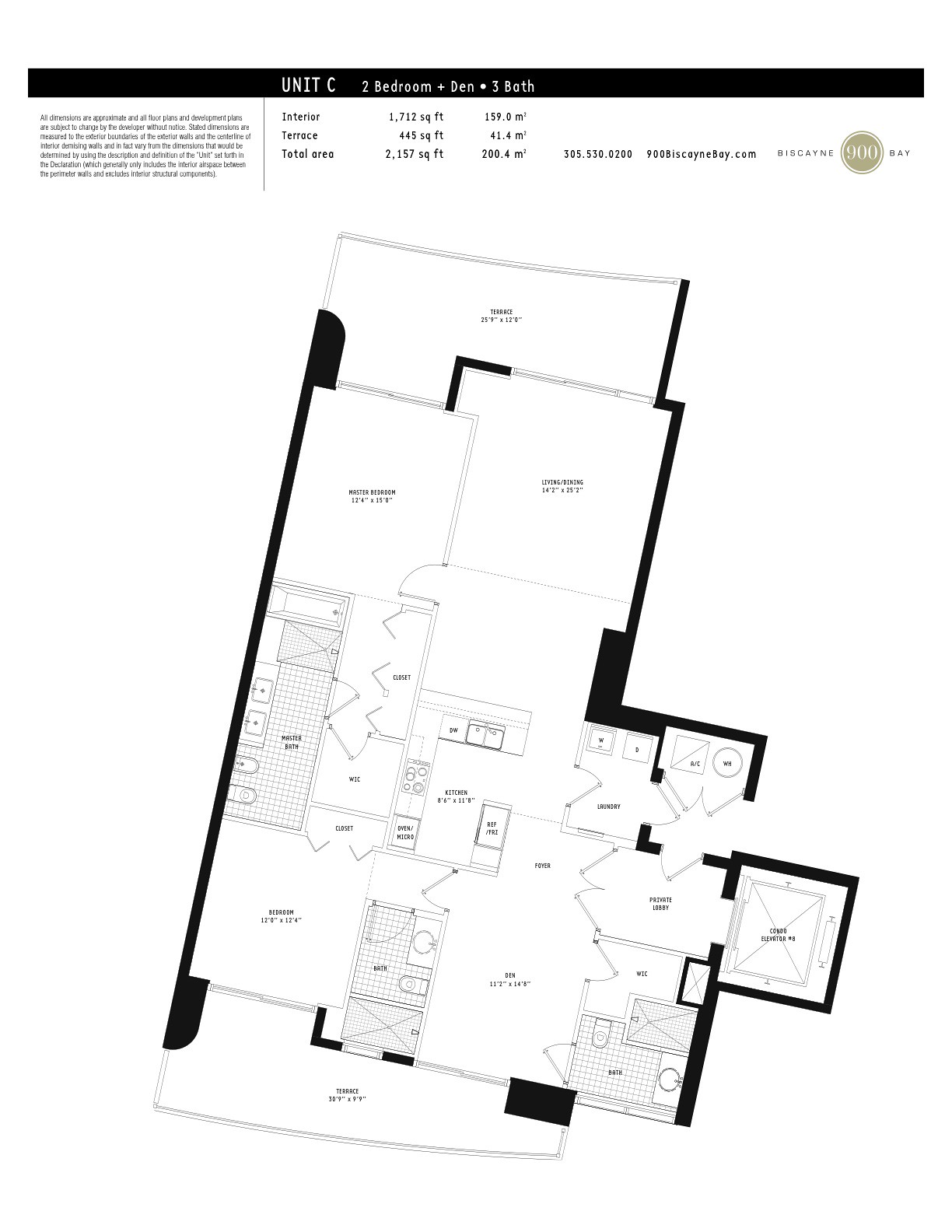**Detailed Caption:**

This detailed floor plan illustrates a luxurious apartment unit identified as "Unit C" which includes two bedrooms, a den, and three bathrooms. At the top of the image, a prominent black bar with white text provides this identification. Just below, a disclaimer in black text on a white background specifies that all dimensions are approximate. 

In the top left corner, a block of text extends various details about the apartment, though much of it is too small to discern. The easily readable components reveal that the interior space measures 1,712 square feet (159.0 square meters) with an additional terrace area of 445 square feet (41.4 square meters), culminating in a total area of 2,157 square feet (200.4 square meters). Additionally, contact details including a phone number, 305-530-0200, and a website, 900BiscayneBay.com, are provided along with the Biscayne Bay logo featuring "900" in white letters within concentric circles of light khaki color.

The actual floor plan is displayed beneath this text and is slightly angled from the lower left to the upper right. The top section features a spacious terrace, the master bedroom, and a versatile living and dining area. Accompanying these spaces are various closets, a compact kitchen, and a laundry room. The lower section includes an entryway accessible via an elevator and two additional bedrooms, each boasting its own en suite bathroom. This part of the apartment also includes a second terrace located at the very bottom of the image.